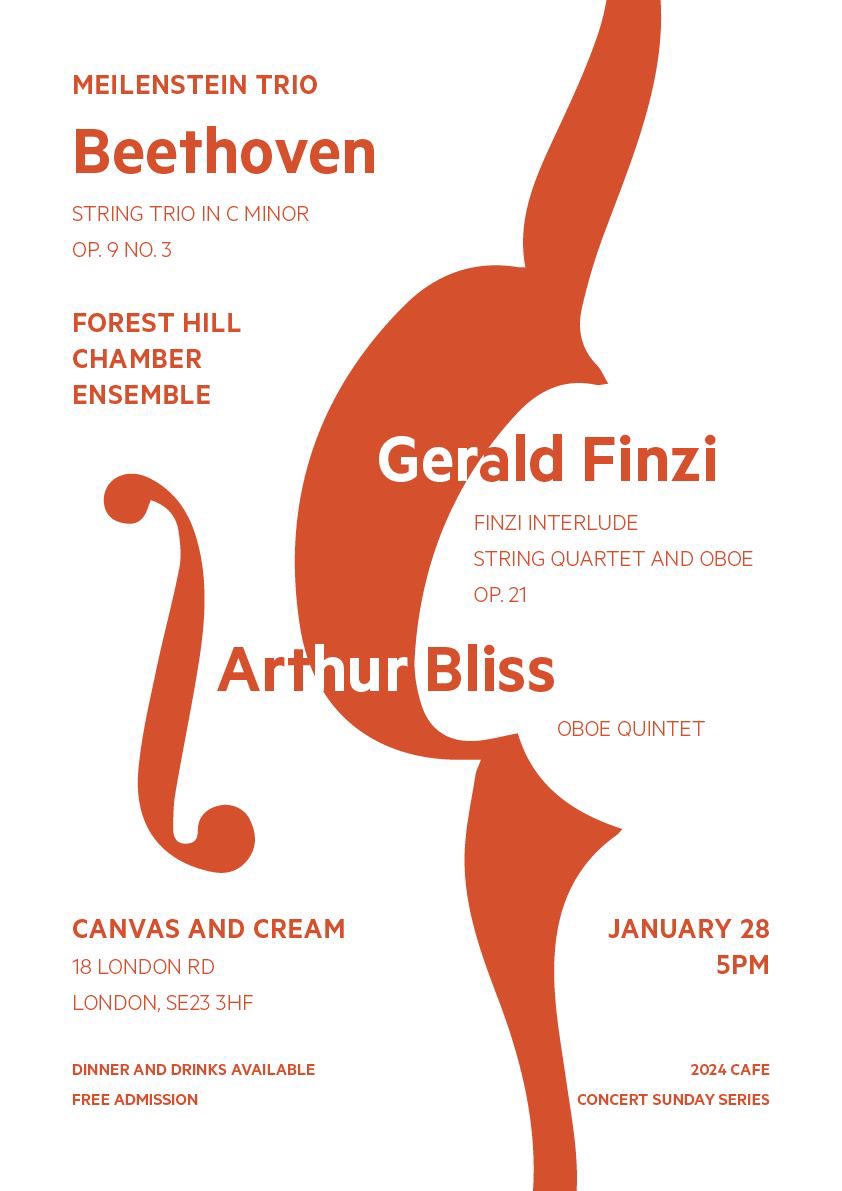This is a meticulously designed digital advertisement for an upcoming musical event. The poster predominantly features a clean, symmetrical layout with a red and white color scheme. Central to the design is an artistic rendering of a musical note in red, extending vertically through the poster and providing a striking backdrop to the text. 

Highlighted in bold red letters are the details of the event: "Nielenstein Trio" performing Beethoven's "String Trio in C Minor, Op. 9 No. 3," hosted by the Forest Hill Chamber Ensemble. The poster also prominently features the names of other performers: Gerald Finzi, known for his String Quartet and Oboe piece, Op. 21, and Arthur Bliss, who will present his Oboe Quintet.

The venue for this musical evening is Canvas and Cream, located at 18 London Road, London, SC 23 3HF. The event is scheduled for January 28th at 5 p.m. as part of the 2024 Cafe Concert Sunday Series. Attendees will enjoy free admission along with dinner and drinks available for purchase.